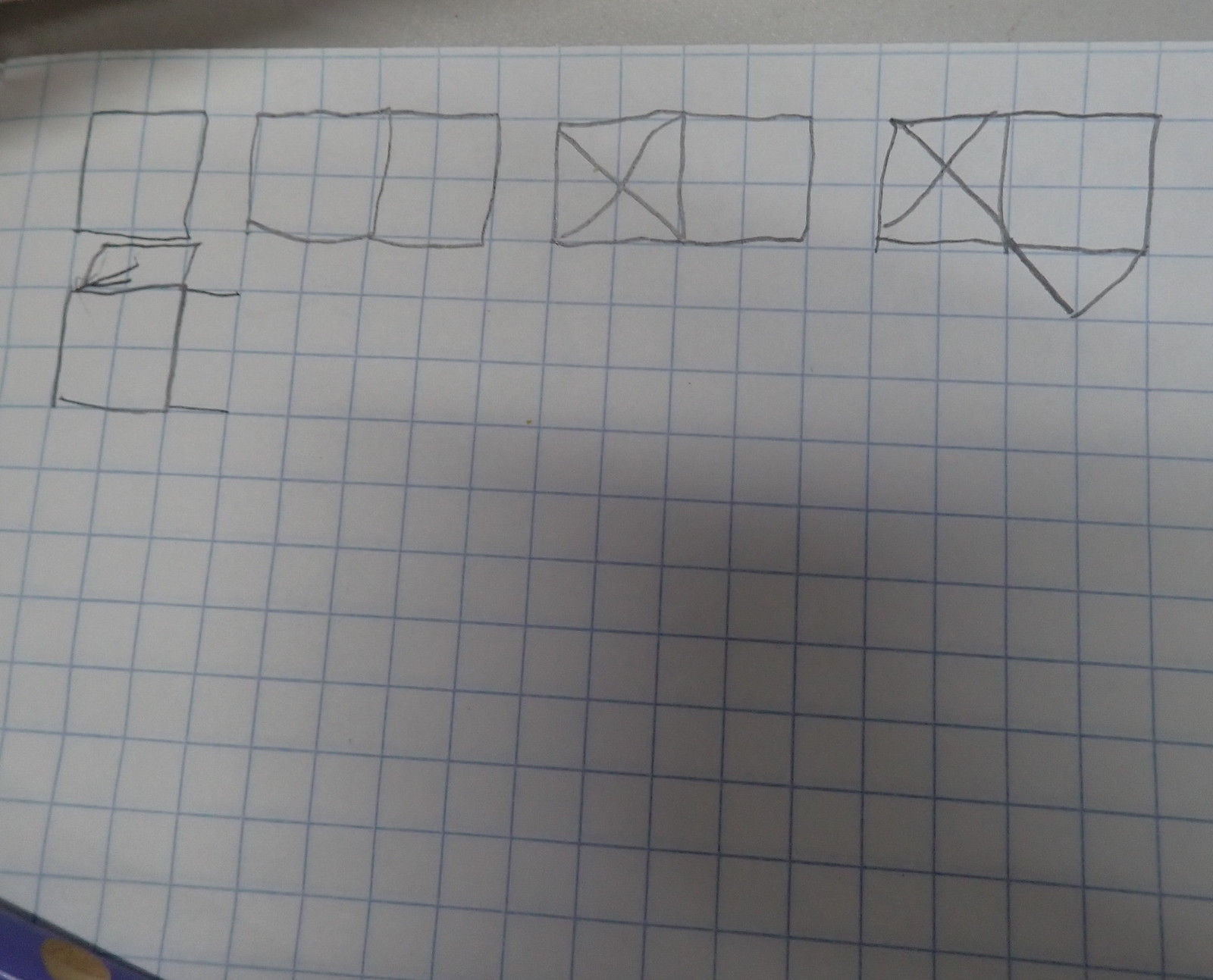A close-up photograph of a rectangular section of white graph paper, slightly wider than it is tall, fills the frame. The image captures approximately half of the graph paper, revealing its light blue grid lines forming small squares. In the lower left corner, a tiny sliver of an indeterminate object—possibly blue or gold—peeks into the frame. At the very top of the image, a thin white strip suggests the edge of a table or the surface the graph paper rests on.

On the graph paper, someone has sketched a series of patterns using the grid. Starting from the upper left, there is a four-square cluster, followed by two more adjacent clusters of the same size. Next, another pair of four-square clusters appears, one of which has an X marked in the left square. In the final cluster to the right, the left square also contains an X, and the right square is intersected by a small triangle at the bottom.

Beneath these clusters, towards the left, there's another four-square cluster. It features two lines extending to the left from the top and bottom squares. Additionally, there is a small pencil lead marking on top of it, with several lines radiating from the lower left quadrant of the cluster.